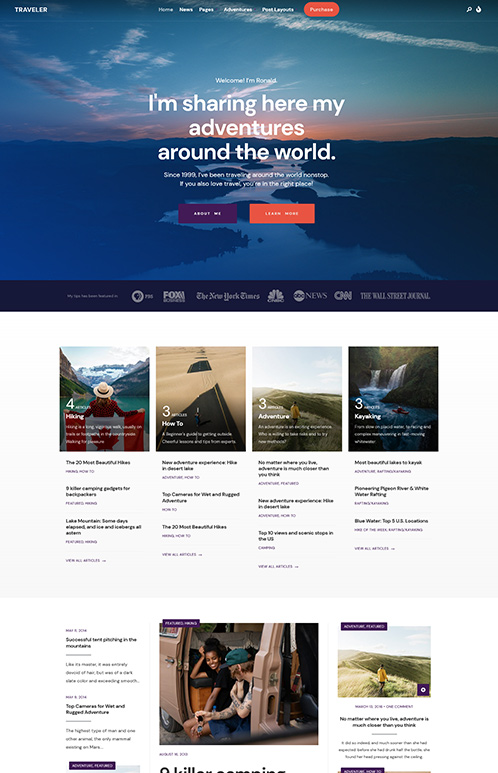The image showcases a travel-themed website with a user-friendly interface. In the top left corner, the word "Travel" is prominently displayed. The navigation bar at the top includes tabs labeled "Home," "News," "Pages," "Adventures," and "Post Layouts," along with an orange "Purchase" button. Although the text appears small and somewhat hard to read, the layout suggests an organized and visually appealing design.

The central area features a captivating landscape image of a river meandering through a dense forest, set against a backdrop of a blue sky tinged with the warm hues of sunset. The positioning of the sun suggests it's late afternoon, casting an orange glow across the scene. Overlaid on the image is a white text that reads, "I'm sharing here my adventures around the world." Beneath this, additional text is present but difficult to decipher.

Below the main image, the website displays logos of prominent news organizations such as The New York Times, Fox News, ABC News, CNN, and The Wall Street Journal, implying the site's recognition or affiliations.

Further down, the website features categorized images, each accompanied by a number indicating the count of related articles. Categories include:
- Hiking (4 articles) with an image of a woman in outdoor gear.
- How-To (3 articles) with a picture showcasing a road, symbolizing guidance or a journey.
- Adventure (3 articles) displaying a person standing in an outdoor setting.
- Kayaking (3 articles) featuring an individual kayaking on a body of water.

Additionally, there's a section with more text and a few more pictures set against a white background, providing further content and visual interest to the page. The overall design aims to inspire and inform visitors about various travel adventures and activities.